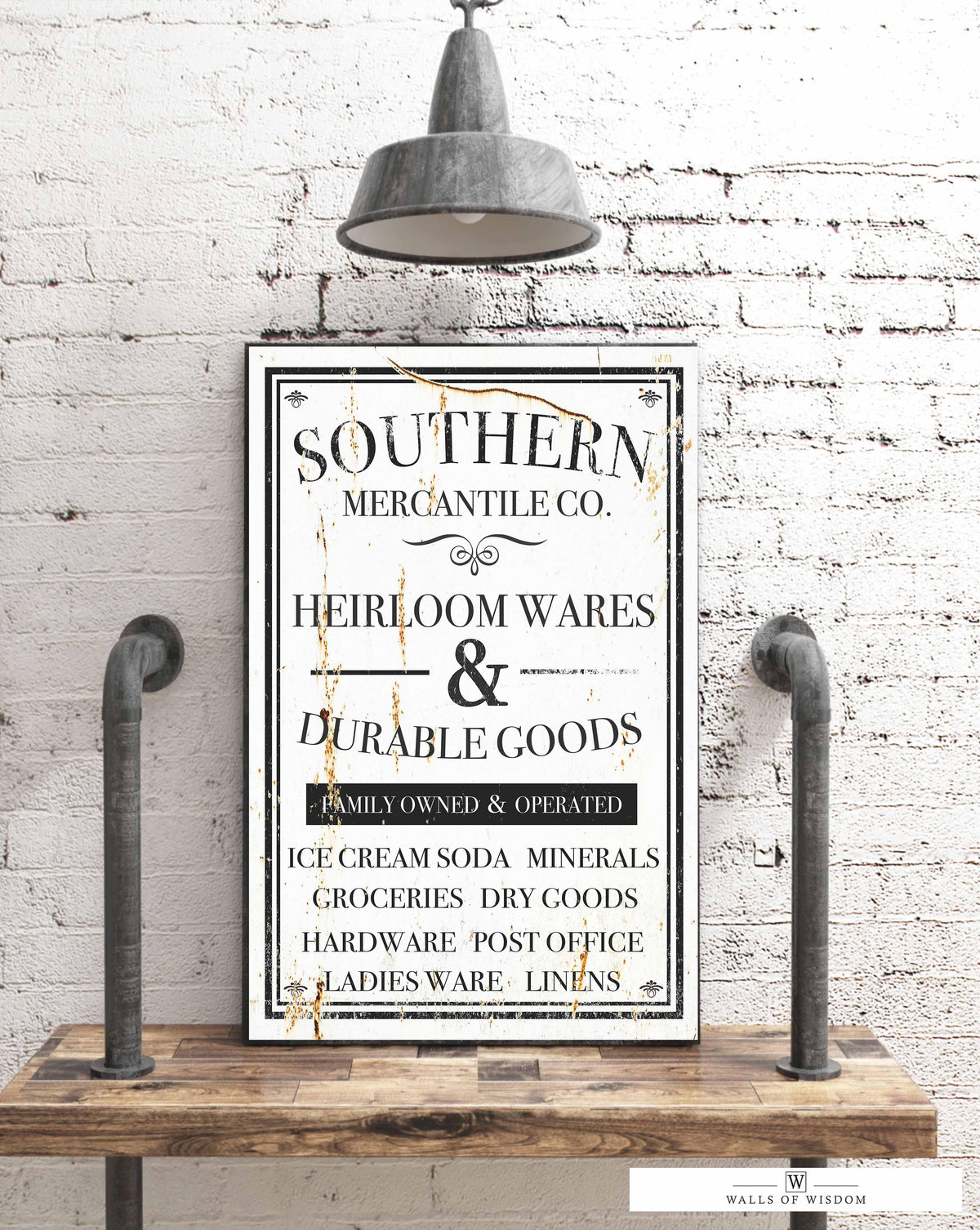The image is a color photograph in portrait orientation, depicting a vintage sign centrally placed against a white brick wall. The sign, which has a slightly worn, antique appearance, is mounted on a brown wooden shelf held up by two black metal pipes on either side. Above the sign, a single bulb lamp with a black metal shade extends from the ceiling, casting light onto the sign.

The sign itself features various texts divided into several sections. At the top, in slightly arched black letters, it reads "Southern Mercantile Co." Below this, in a script flourish, are the words "Heirloom Wares and Durable Goods." Further down, on a black horizontal strip with white text, it states "Family Owned and Operated." The lower portion of the sign lists a variety of goods and services offered by the establishment, including "ice cream, soda, minerals, groceries, dry goods, hardware, post office, ladies wear, and linens." The sign also features random rust marks, adding to its antique charm. The entire arrangement is a visual representation of a bygone era, possibly from the late 1800s, radiating a nostalgic ambiance. On the bottom right corner of the sign, there is a small white strip with a black logo, "W," followed by the words "Walls of Wisdom."